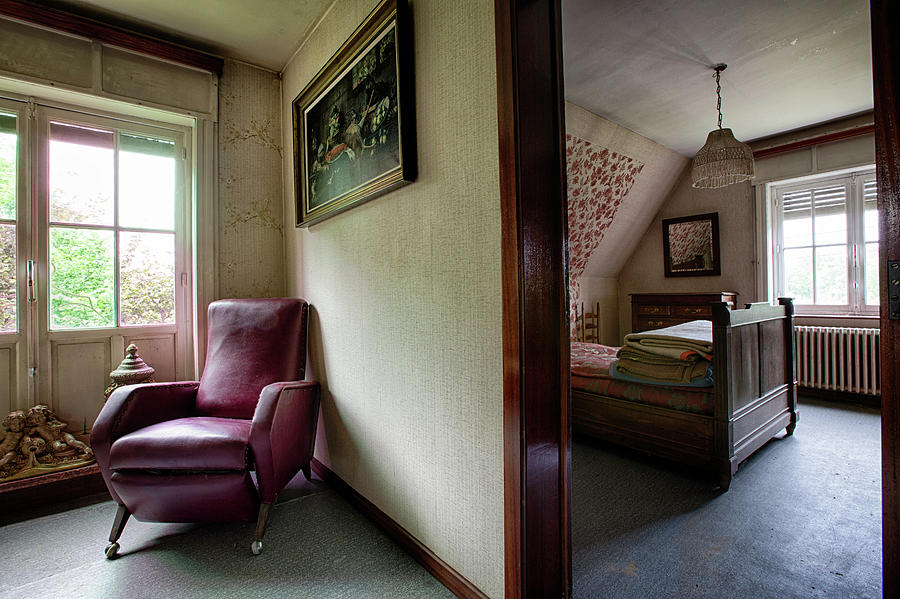The image depicts the interior of an old-timey house, captured from the center of a doorway, providing a view into both a living room and a bedroom. The left room, the living room, features two wide windows with light shades, revealing a view of the yard with some trees. Below the windows are statues of two cherubs and an urn. A maroon seating chair, resembling a recliner but stationary, is situated in the corner next to the windows. On the adjacent wall hangs a dark painting with a gold frame, set against light beige walls. 

The right room, the bedroom, contains a dark brown wooden bed, topped with neatly folded blankets. A chandelier hangs centrally from the ceiling, adding a touch of elegance. Beneath another set of windows, which may double as doors leading outside, are room heaters. The walls are adorned with wallpaper, and a mirror is hung at the back of the room, reflecting the decorative elements.